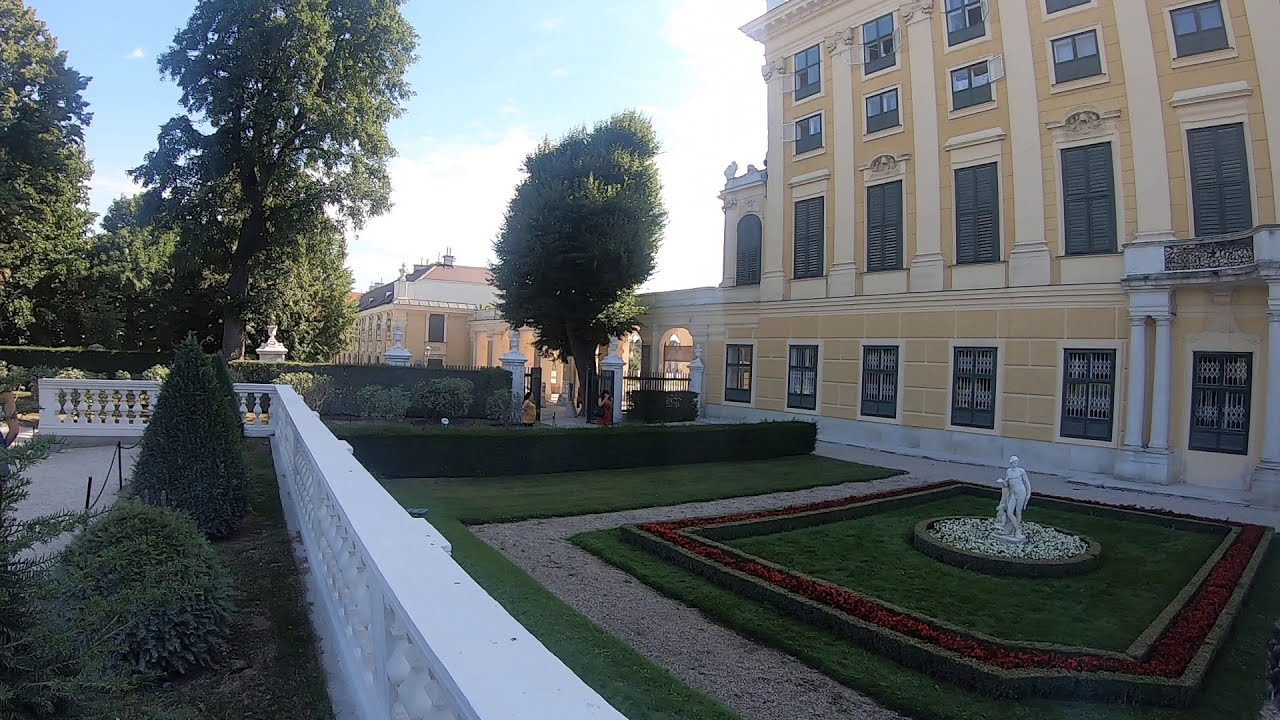The image illustrates an outdoor scene of a meticulously maintained garden or courtyard adjacent to a luxurious multi-story yellow stone building with numerous black windows, exuding an upper-class elegance. The building, which spans roughly half of the picture, is connected to a similar structure in the background via a covered walkway, held up by arched pillars. This courtyard, defined by manicured grass, a hedge, and a decorative pathway forming a square, features a central grassy area bordered by red flowers and a circular rock garden with a classical white marble statue, possibly depicting a woman, at its heart. To the near side of the courtyard is a white decorative fence, and in the foreground, there's a bed of evergreen shrubs alongside the white wall with small pillars. The setting could be a high-end hotel, an upscale resort, or a prestigious college building, characterized by its luxury and attention to detail, including the presence of tall trees and possibly two women in the background.